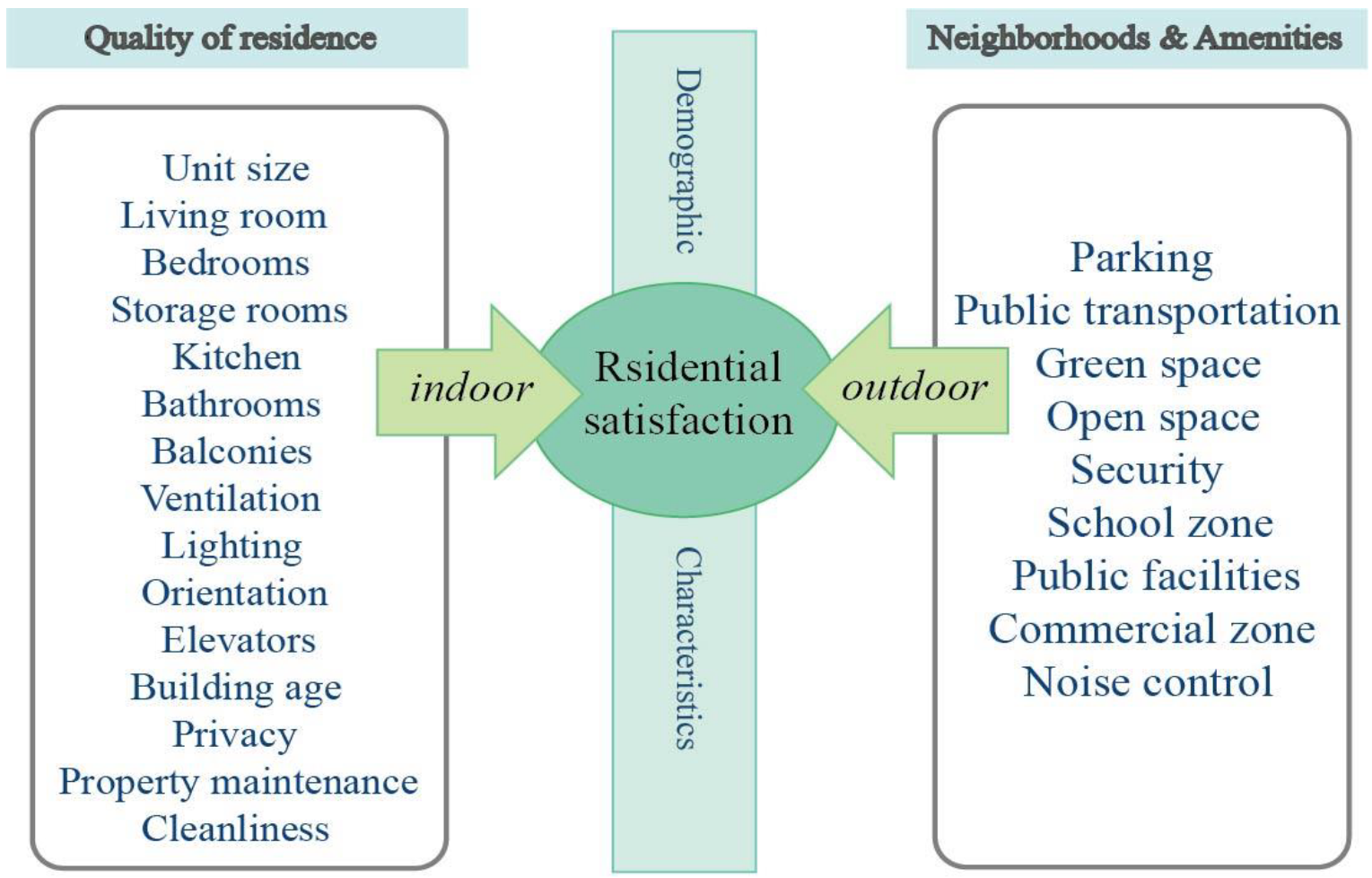The image is an informational diagram that illustrates the factors contributing to residential satisfaction. It features two columns on either side of a central circle. The left column, titled "Quality of Residence," lists indoor attributes such as unit size, living room, bedrooms, storage rooms, kitchens, bathrooms, balconies, ventilation, lighting, orientation, elevators, building age, privacy, property maintenance, and cleanliness. An arrow labeled "Indoor" points from this list to the central circle. 

The right column is labeled "Neighborhoods and Amenities" and includes outdoor features like parking, public transportation, green space, open space, security, school zone, public facilities, commercial zone, and noise control. An arrow labeled "Outdoor" directs from this list to the central circle. The image emphasizes that both indoor and outdoor variables affect "Residential Satisfaction," represented by the circle in the middle. Additionally, a vertical label, "Demographic Characteristics," runs through the center, suggesting the influence of demographic factors on residential satisfaction.